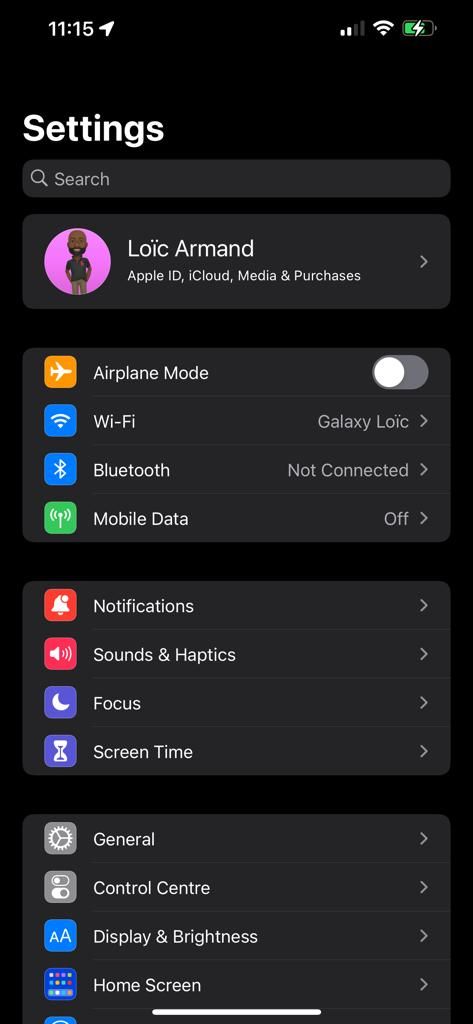The image displays the Settings page of an Apple smartphone against a black background. At the top left, the word "Settings" is written in white. Below "Settings" is a search box labeled "Search". Beneath the search box, there is a user profile belonging to "Loic Amand," with the accompanying text "Apple ID, iCloud, Media & Purchases". To the left of the user name, there is a pink profile icon featuring a character with a black beard, wearing a black t-shirt and brown trousers.

Below the profile section, there is a settings category that includes several options:
- **Airplane Mode**: Off
- **Wi-Fi**: Connected to Galaxy_Loic
- **Bluetooth**: Not Connected
- **Mobile Data**: Off

Following this, another section houses four additional settings:
- **Notifications**
- **Sounds & Haptics**
- **Focus**
- **Screen Time**

At the bottom is a larger section containing more settings:
- **General**
- **Control Center**
- **Display & Brightness**
- **Home Screen**
- **Additional options**

Each of these settings options is accompanied by an icon on the left side. These icons vary in color, including blue, green, orange, purple, grey, and yellow for Airplane Mode.